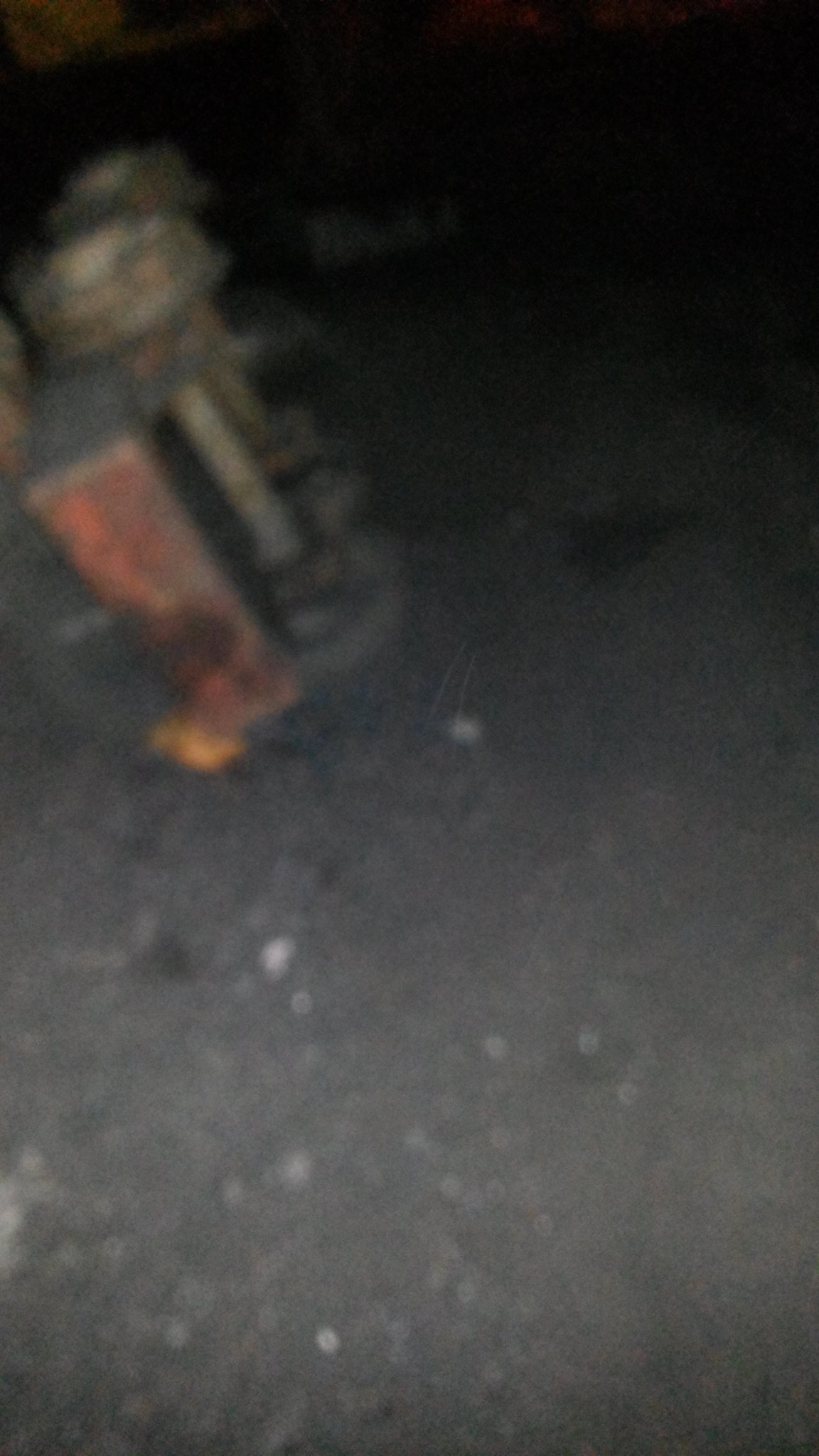In the image, there is a very blurry and grainy scene taken outdoors or possibly in a garage, with a dirt or concrete floor. The photo, captured at what appears to be sundown with a flash, shows a dark, gray environment with some small white particles floating around due to the flash reflecting off the dust. At the center-left of the image, there is a rectangular-shaped object with an orange and yellow side, which seems to be a machine or a tool. The device has several metal components, including a tube in the center and another tube extending to a square metal part at the front. In the background, there are vague outlines that might be a tree or other elements of the surroundings, but due to the poor quality and significant blur of the photo, the exact details are indistinct and difficult to determine.